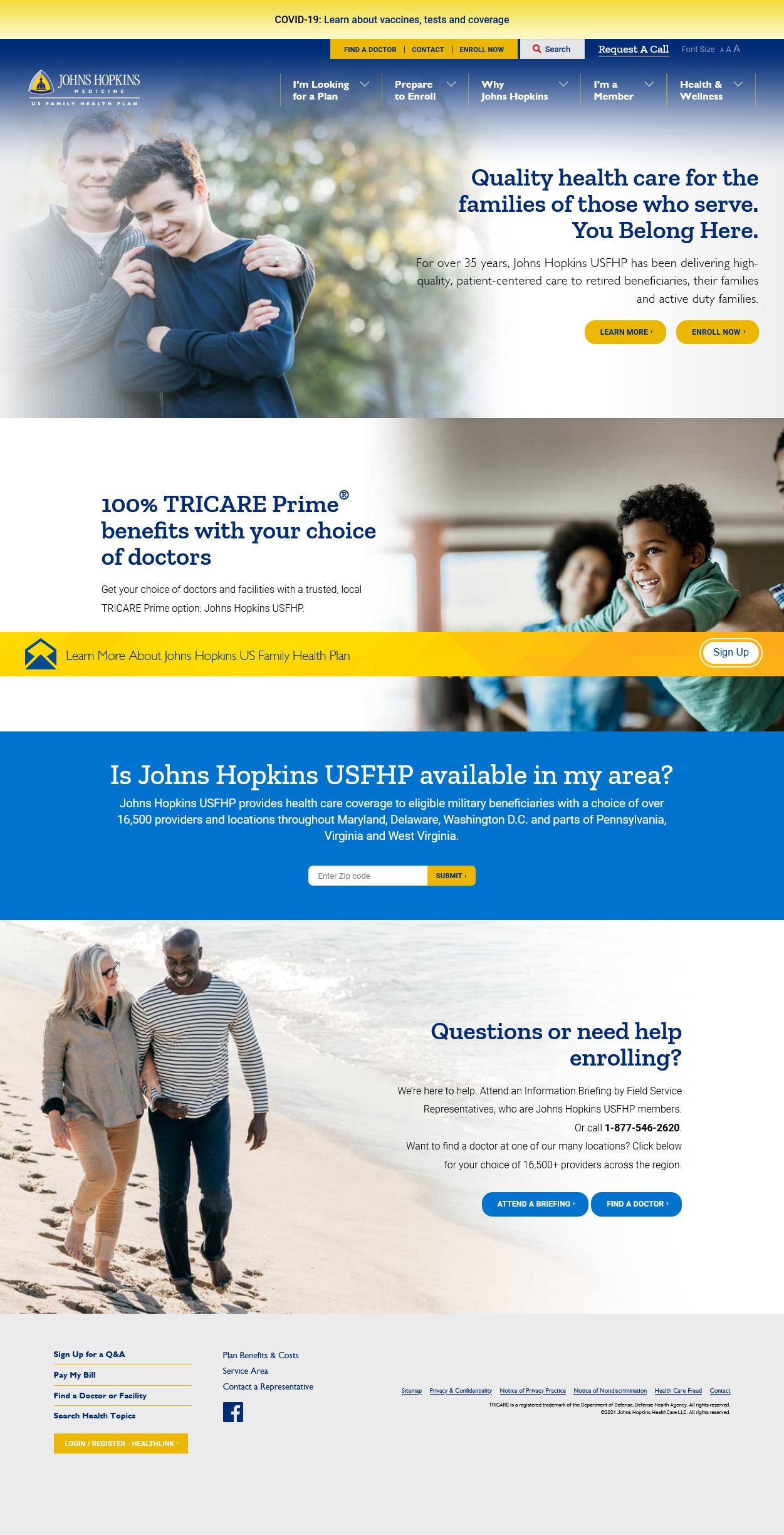This is a detailed caption for an image depicting a healthcare facility's website:

---

**Screenshot of the Johns Hopkins Medicine Family Health Plan Website**

At the top of the website, there is a prominent banner addressing COVID-19, with options to learn about vaccines, tests, and coverage. The upper left corner features the Johns Hopkins Medicine logo, accompanied by the text "Family Health Plan."

Various navigational options are displayed: "Find a Doctor," "Contact," "Enroll Now," "Search," and "Request a Call." Additional user-centric links include "I'm Looking for a Plan," "Prepare to Enroll," "Why Johns Hopkins," "I'm a Member," and "Health and Wellness."

Central to the page is a heartfelt image of a family: an older man, presumably the teenager's father, standing next to him, and a middle-aged man affectionately holding his young teenage son by the shoulders. Behind them, a serene backdrop of trees is visible.

To the right of this family image, a compelling message reads: "Quality healthcare for the families of those who serve. You belong here. For over 35 years, Johns Hopkins USFHP has been delivering high-quality, patient-centered care to retired beneficiaries, their families, and active-duty families. Learn more and enroll now."

The remainder of the page contains additional information, led by a headline declaring: "100% TRICARE Prime benefits with your choice of doctors." A prompt follows, encouraging visitors to "Learn more about Johns Hopkins US Family Health Plan" and check if "Johns Hopkins USFHP is available in my area."

Below this text, another image features a man and a woman joyfully walking on a beach. To the right of this image, a support message states: "Questions or need help enrolling? We're here to help. Attend an information briefing by field service representatives who are Johns Hopkins USFHP members."

This comprehensive online resource invites users to join a community dedicated to high-quality, accessible healthcare.